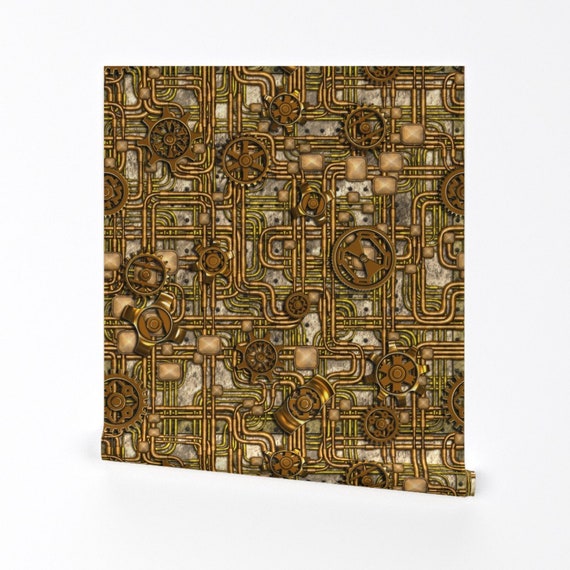The image features a detailed design resembling an intricate, ancient machine spread out against a monochromatic, silver background. The main pattern is composed of a complex array of interwoven brass and gold-colored tubes and pipes, some paired and others running solo, connected by a series of gears and circular shapes. These gears vary widely in style and detail, some with six spokes and differing centers, showcasing a rich, dark bronze hue. At the bottom of the image, the design seems to be rolling up like a piece of paper or fabric, giving the sense that it’s either wallpaper or some type of wrapping paper, accentuating how the elaborate mechanics-like design fades into the background.